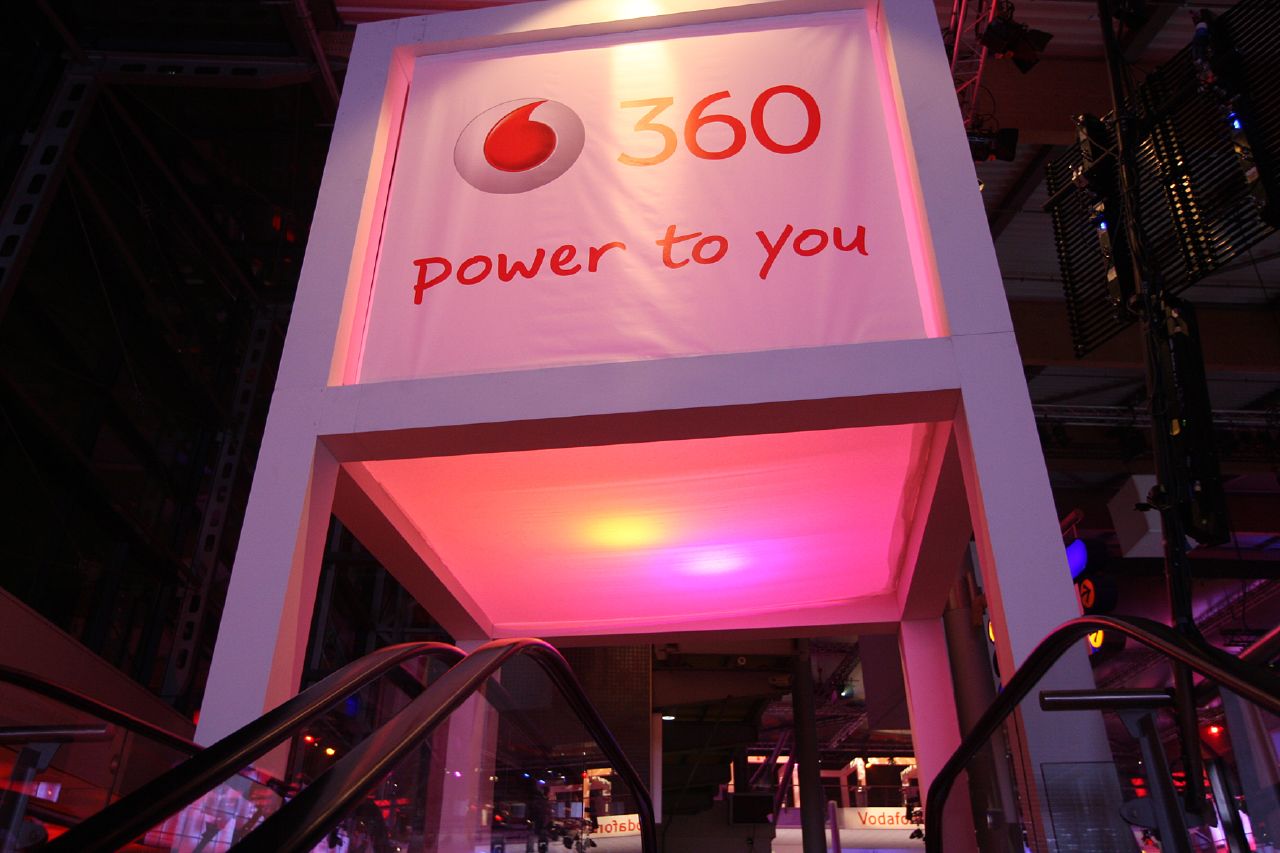The image captures the top section of an escalator in a dimly lit indoor setting, possibly within a mall or similar environment. Central to the composition is a prominent fixture, approximately 20 feet high, supported by four white legs. The fixture features a large sign that reads "360 power to you" in bold red letters against a white background. To the left of the text is a white circle with a red teardrop symbol. The underside of the sign is illuminated with yellow lighting, diffused through a pink, semi-transparent panel, likely made of plexiglass. This illuminated area casts a glowing effect on the scene below.

The foreground reveals two guardrails leading to or from the escalator, while the background shows a mix of dark and lit areas, hinting at various store signs and the high, metallic, and black-beamed ceiling above. A few people are visible, scattered in the distance, suggesting light foot traffic within this spacious, bustling environment.